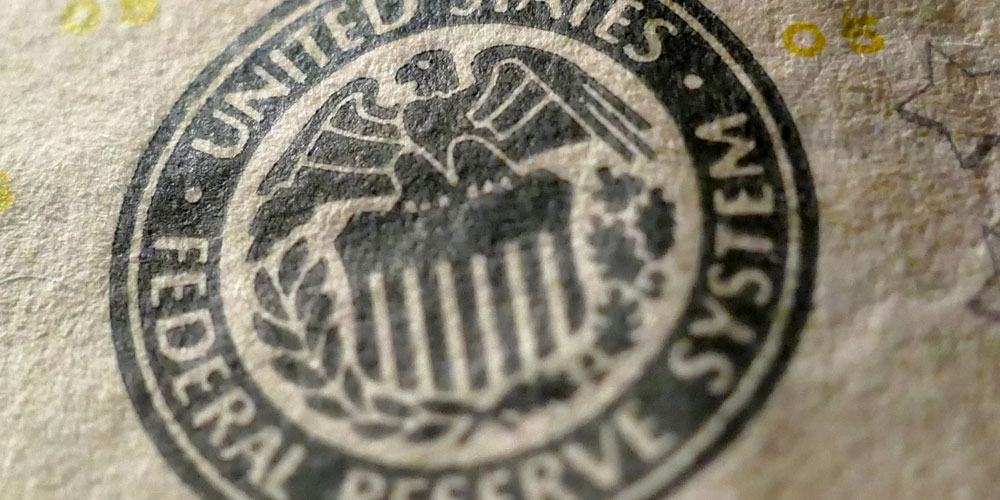The image showcases the emblem of the United States Federal Reserve System. Central to the emblem is a majestic eagle with its wings spread, positioned above what appears to be a pillared structure. Beneath the eagle, a wreath combines laurel and oak leaves, extending upwards from the bottom edges of the circular design, creating a semi-circular frame around the eagle. The emblem contains the words "United States Federal Reserve System" inscribed along the outer ring of the circle, directly following the curve. The emblem is printed in black ink on a tan, textured surface, possibly paper, exhibiting occasional yellowish spots in the upper left, upper right, and left side areas. There are also hand-drawn stars visible in the vicinity of the right corner and side. Additionally, numbers "0" and "6" appear next to the emblem, hinting at its potential connection to currency or a type of bill.